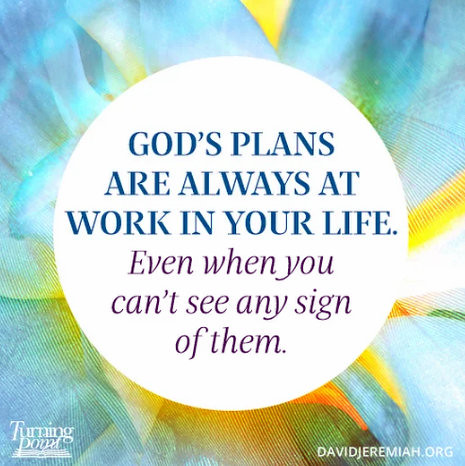The image features an abstract, multi-colored background with swirls and swashes of blue, yellow, and white. Prominently centered in the image is a large white oval, serving as a canvas for a motivational message. At the top of the oval, bold blue, uppercase text declares, "God's plans are always at work in your life." Directly beneath this, in purple italicized lowercase text, it continues, "even when you can't see any sign of them." In the lower left corner of the image, there is a white logo for Turning Point Ministries, while the lower right corner displays the text "DavidJeremiah.org" in white, linking the inspirational message to its source.